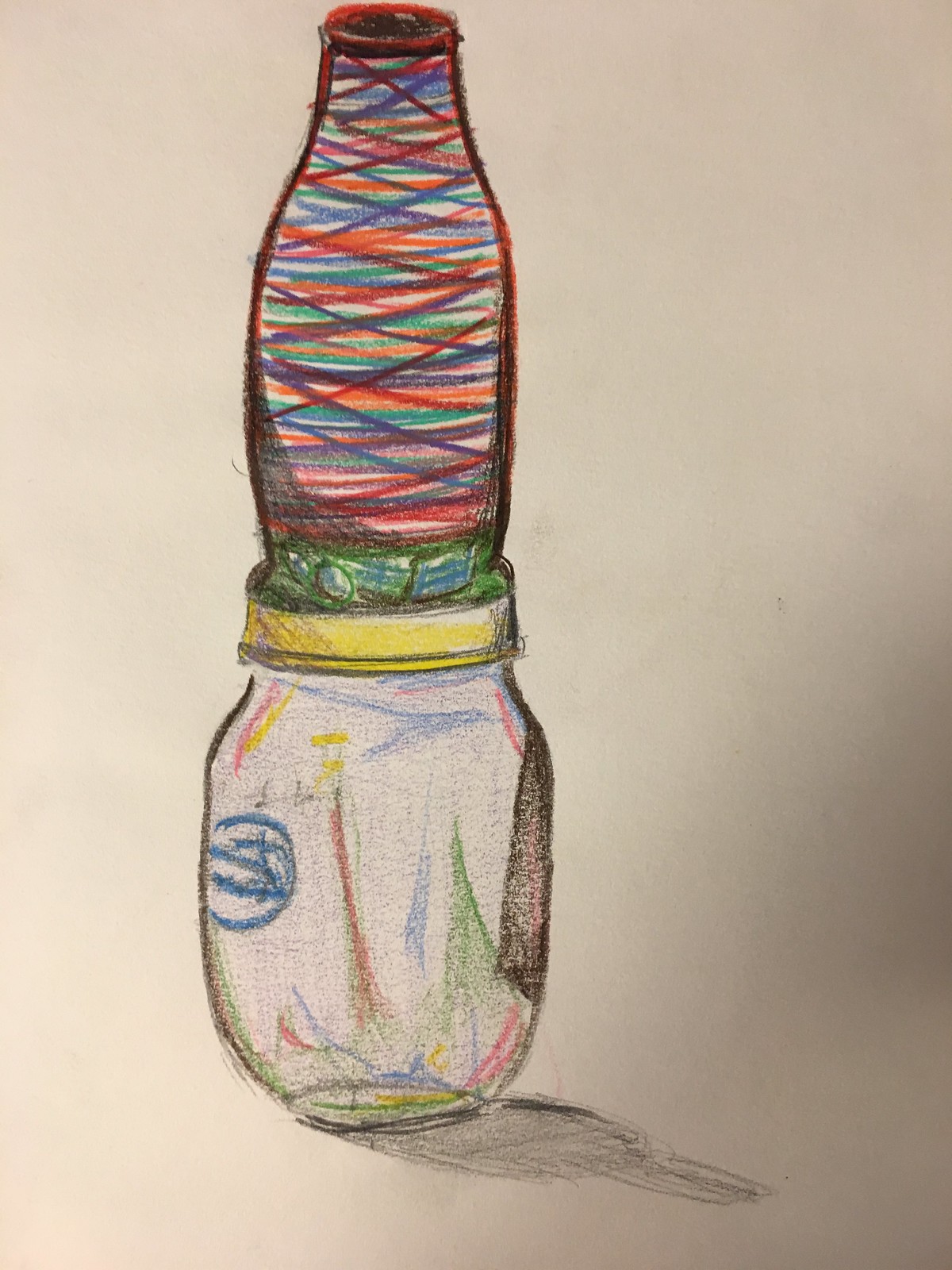This image showcases a highly detailed sketch, likely created with colored pencils due to the precision of the lines. At the base of the drawing, there is an intricately designed, transparent jar adorned with vibrant, crisscrossing lines in shades of red, green, yellow, blue, and black. Careful attention has been given to the jar's shadow, which extends to the right and is rendered in a soft graphite pencil. Attached to the top of the jar is a striking, bottle-like structure. It is beautifully colorful, featuring an array of blue, orange, green, and red lines in a crosshatched pattern from the base to the tapered top. The base of the bottle begins in green, narrowing upwards to meet a distinct bottle cap. The entire composition is unified as a single, coherent piece, displaying a rich tapestry of color and detail.